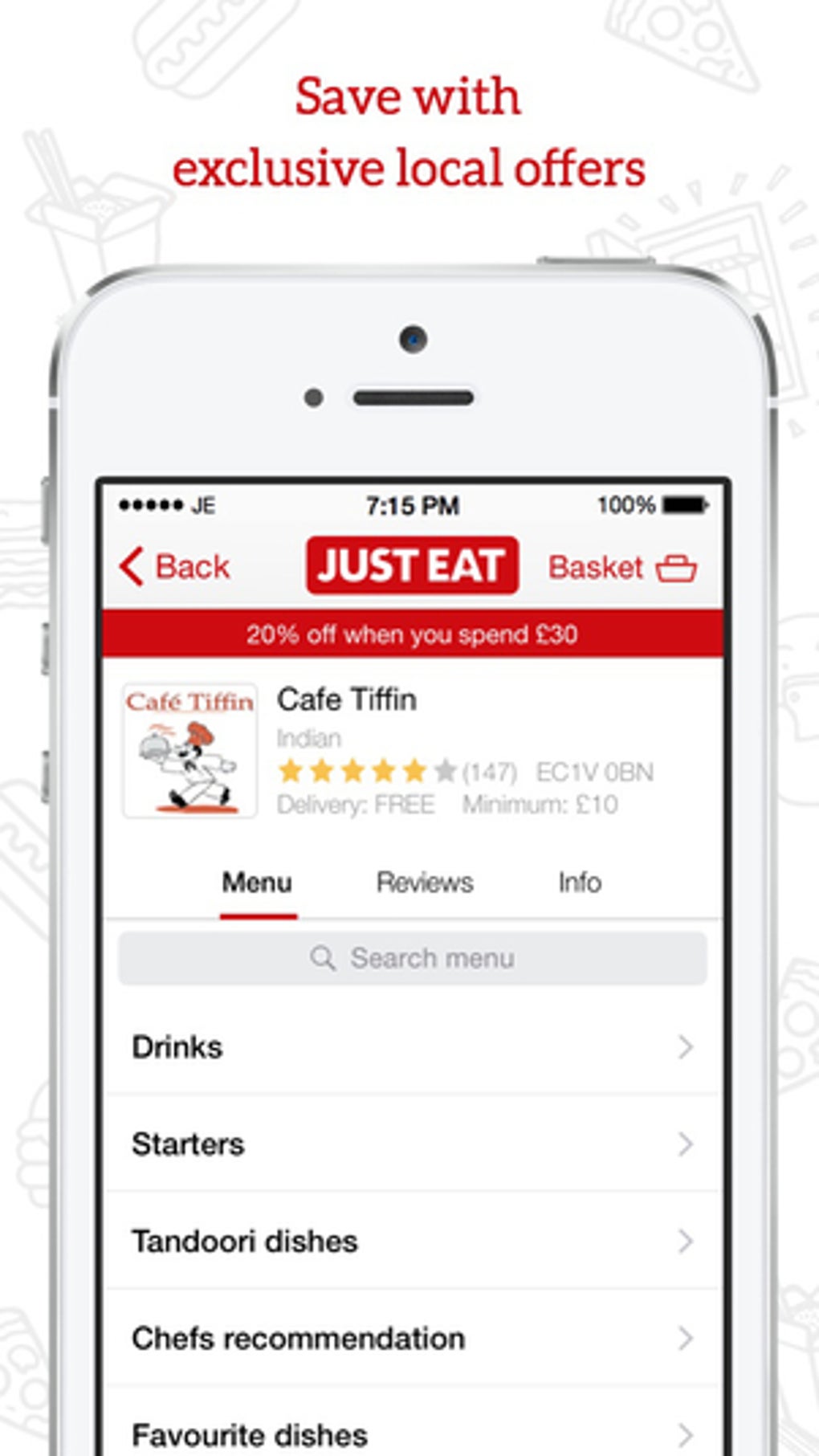The image depicts an advertisement featuring an iPhone at its center. The background is predominantly white, adorned with subtle gray icons representing various food items. At the top of the advertisement, bold red text announces, "Save with Exclusive Local Offers."

The iPhone displayed in the middle showcases a mobile application screen. At the top of the screen, the status bar indicates the time as 7:15, a fully charged battery, and maximum signal strength. Below this, a prominent red button with white text reads “Just Eat.” Adjacent to this button, navigation icons for 'Back' and 'Basket' are visible.

Directly under these elements, a promotional message declares, "20% off when you spend 30 euros or pounds." Beneath this, there is an icon for "Cafe Tiffin," which features a cartoon depiction of a chef holding food. The restaurant is denoted as an Indian establishment and boasts a rating of five out of six stars, based on 147 reviews.

The app interface includes a highlighted menu option showcasing categories such as Drinks, Starters, Tandoori Dishes, Chef's Recommendation, and Favorite Dishes. Additionally, tabs for Reviews and Info are present, offering further details about the restaurant and customer feedback.